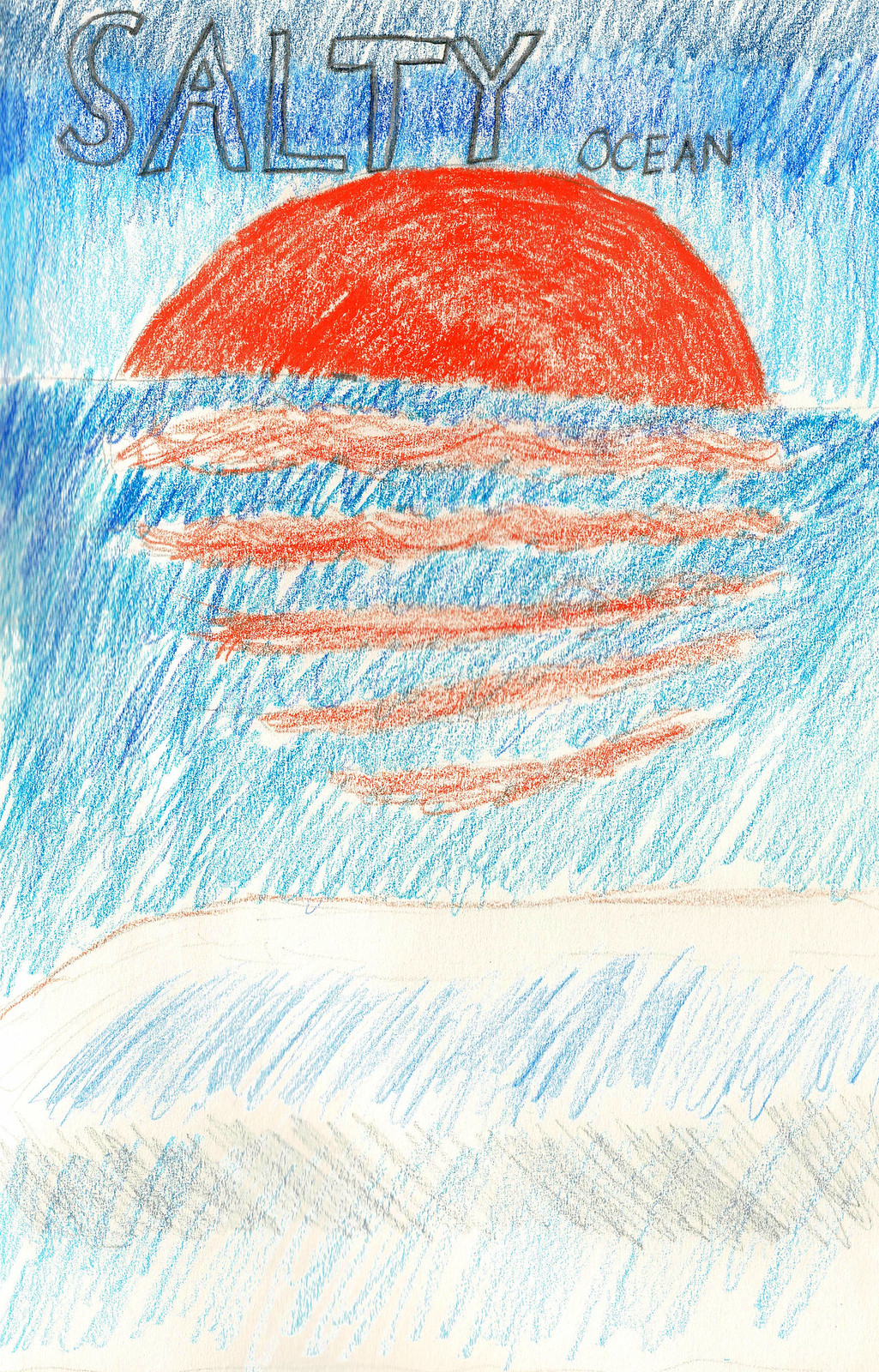The image depicts a hand-drawn illustration that appears to be the work of a child, characterized by its vibrant yet somewhat messy coloring. The entire background is filled with various shades of blue, scribbled broadly yet fully, without any visible edges of the paper. This creates a chaotic but complete backdrop.

At the top left of the illustration, the word "SALTY" is inscribed in large, bold, black capital letters, followed by the word "OCEAN" in a smaller but similarly capitalized format. Below this text, an irregular red half-circle, presumably the sun, dominates the sky, suggesting it is either setting or rising.

Beneath the sun, the ocean is depicted with more squiggly lines in different hues of blue. Amidst these blue lines, sporadic red squiggles represent the sun's reflection on the water, enhancing the sunset theme. Further down, a brown outline likely symbolizes a coastline, contrasting against the principal sea colors. Lighter blue squiggles over this area suggest waves approaching the shore, blending into what seems to be an off-white or sandy-colored section, portraying a beach.

The overall impression is one of a sunset over the ocean, with imaginative use of color and form that, while messy, evokes a playful and innocent representation of a seascape drawn from a child's perspective.